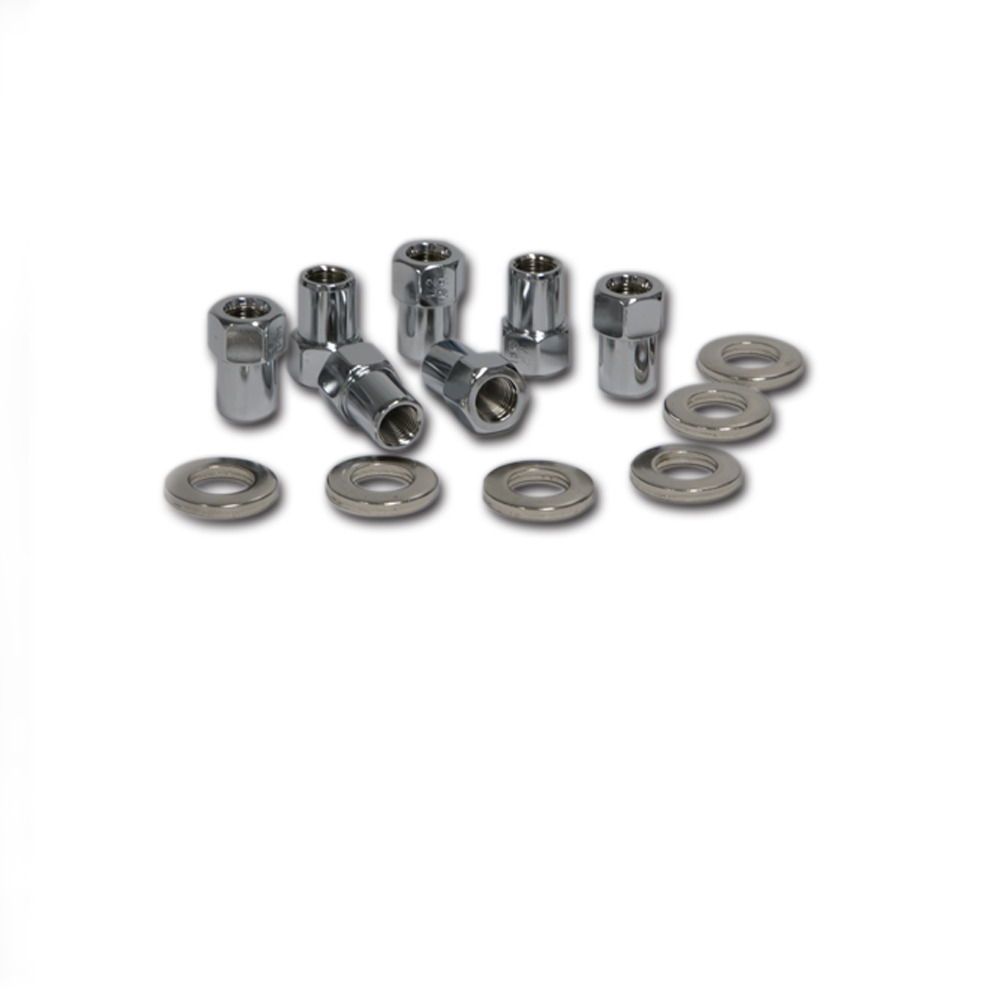The image showcases an assortment of metallic components arranged meticulously on a pristine white background, emphasizing their reflective chrome finish. Dominating the foreground are six gleaming washers, organized in two sets of three—one trio aligned, and the other trio extending diagonally. Just behind the washers, there are seven shiny hexagonal sockets, five of which are standing upright. These sockets feature alternating nut faces and smooth cylindrical extensions, adorned with subtle metal markings. The remaining two sockets lie flat on their sides, one oriented towards the viewer and the other facing away. Each item casts a narrow yet distinct shadow, heightening their three-dimensional presence. The entire layout, with its clean lines and polished surfaces, exudes a sense of precision and newness, typical of a high-quality toolset product shot.